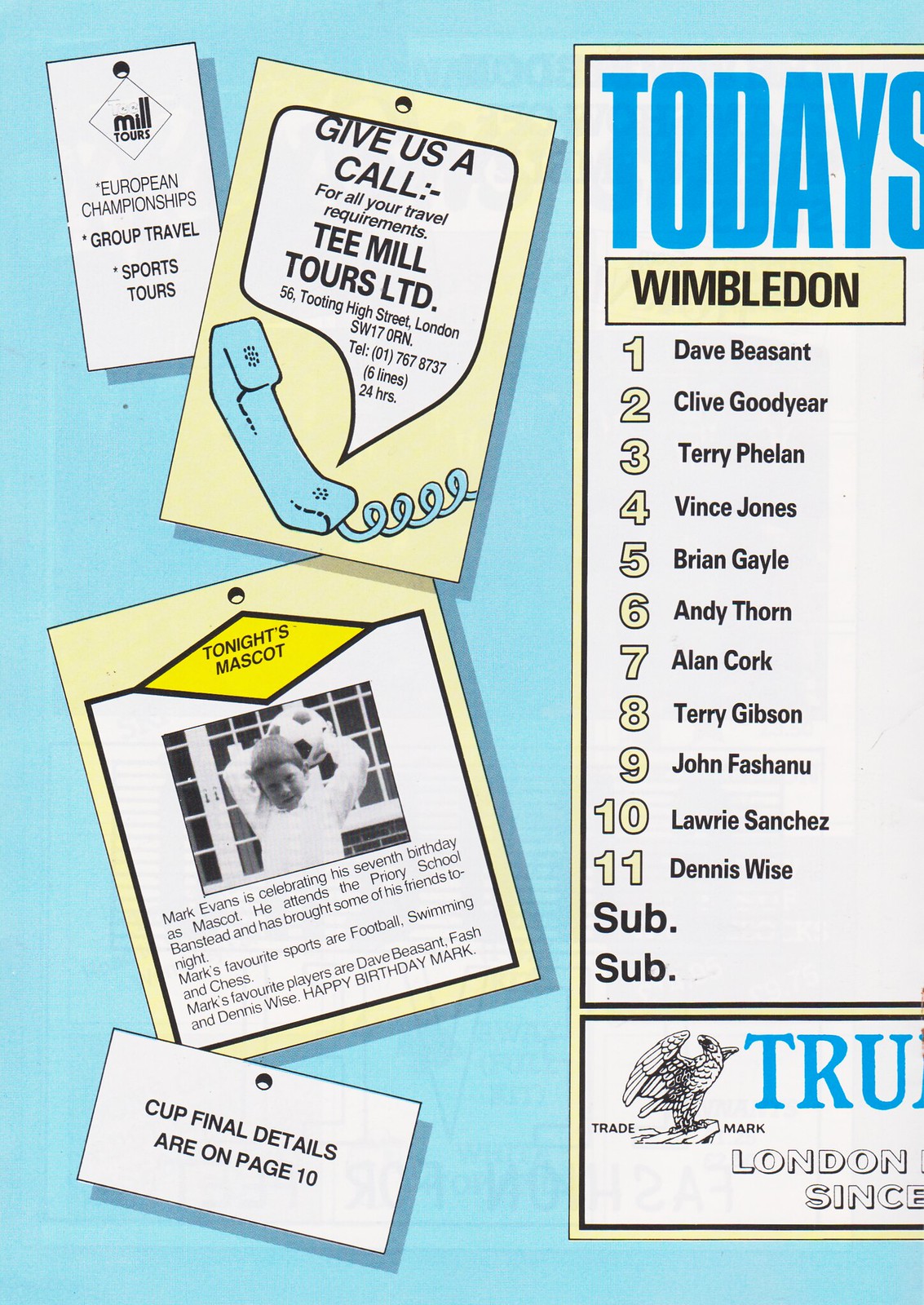The digital poster features a light blue background, occupying about 65% of the image, predominantly on the left-hand side. This section is filled with numerous smaller rectangular-shaped posters and tags. At the very top left, a white poster with black text lists "Mill tours, European Championships, Group Travel, Sports Tour." Below it, another poster reads, "Give us a call for all your travel requirements, T-Mill Tours Limited," accompanied by a drawing of a blue telephone. Further down, on a diamond-shaped yellow background, it announces, "Today's mascot: Mark Evans is celebrating his seventh birthday and attends the Proxy School," with a black and white photo of a smiling child in a white shirt with arms raised. The bottom poster informs that "Cup final details are on page 10."

On the right side of the image, a longer, thinner rectangular bar, partially visible, reads "Today's Wimbledon" in large blue letters at the top, followed by an outlined list of players: 1) Dave Besant, 2) Clive Goodyear, 3) Terry Flawn, 4) Vince Jones, 5) Brian Gale, 6) Andy Thorne, 7) Alan Cook, 8) Terry Gibson, 9) John Fastenew, 10) Laurie Sanchez, and 11) Dennis Wise. Below the list is a logo of a bird, with text mostly cut off, indicating a trademark.